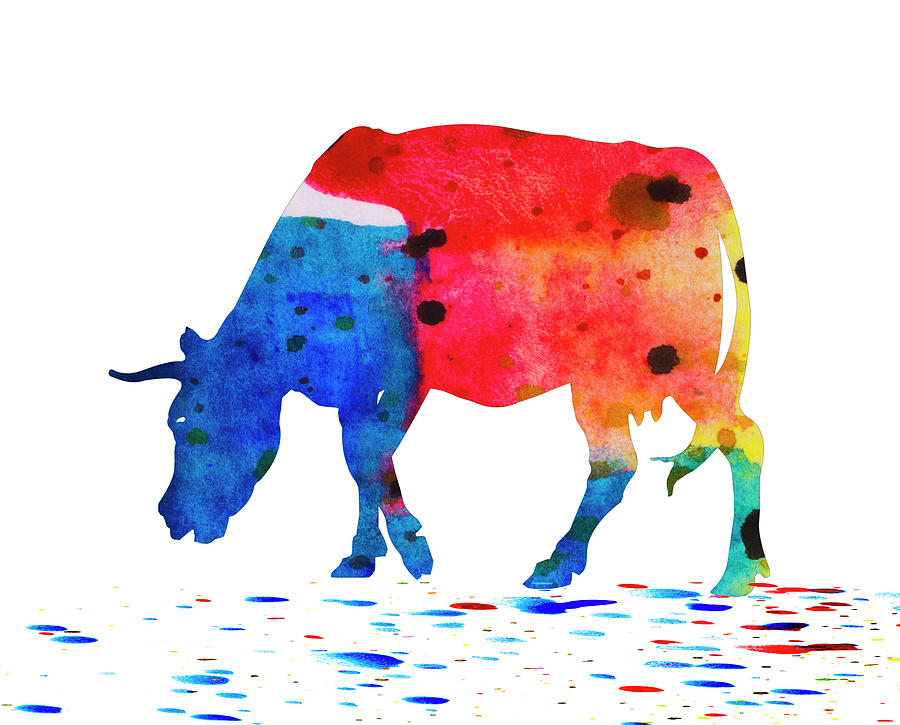This abstract watercolor painting depicts a multicolored cow on a white background, characterized by its vivid and dynamic color palette. The cow’s head, painted in blue, is bent down as if grazing, with its mouth slightly open. From the neck to the shoulders and midsection, the colors transition to a vibrant red, orange, and yellow mix, with dark black and brown spots scattered throughout its body. The front legs are predominantly blue, with one hoof showing a hint of red. The hind legs are a mix of blue and green, flowing into a yellow tail with a teal tip resting on the ground. Surrounding the cow, the ground features an assortment of colorful specks and drops including blue, red, yellow, and green, adding to the painting's lively and textured feel. Despite the clarity of the cow's form, the use of color and speckling details presents a dreamy, somewhat abstract depiction typical of watercolor artistry.